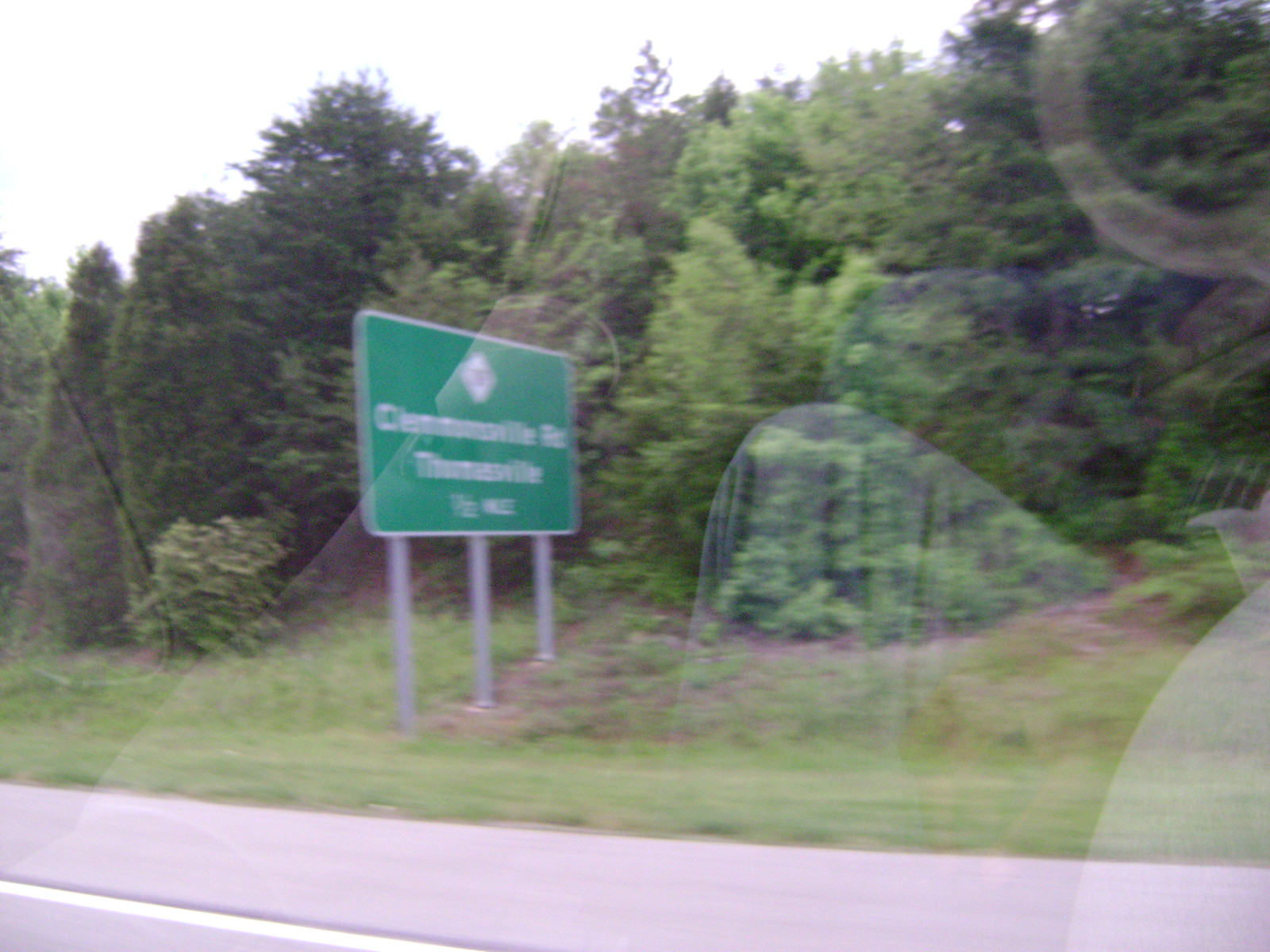This detailed caption incorporates and emphasizes the shared and repeated details from the provided descriptions:

This photograph was taken through the window of a moving car, capturing the outside scenery and reflecting part of the car's interior. The reflection shows the person's bent knee and possibly their hand or pants. The vehicle is moving along a street bordered by a white line marking the shoulder of the road. In the background, a large green rectangular street sign with white writing stands prominently, supported by three metal posts. Behind the sign, the landscape features lush greenery with numerous tall trees, including both coniferous and deciduous varieties as well as smaller shrubs, giving the impression of a dense wooded area possibly on a hillside. The sky above is completely overcast, appearing white in the photograph, suggesting it was taken during the daytime. The road appears to be a multi-lane highway, inferred from the empty lane visible next to the car.